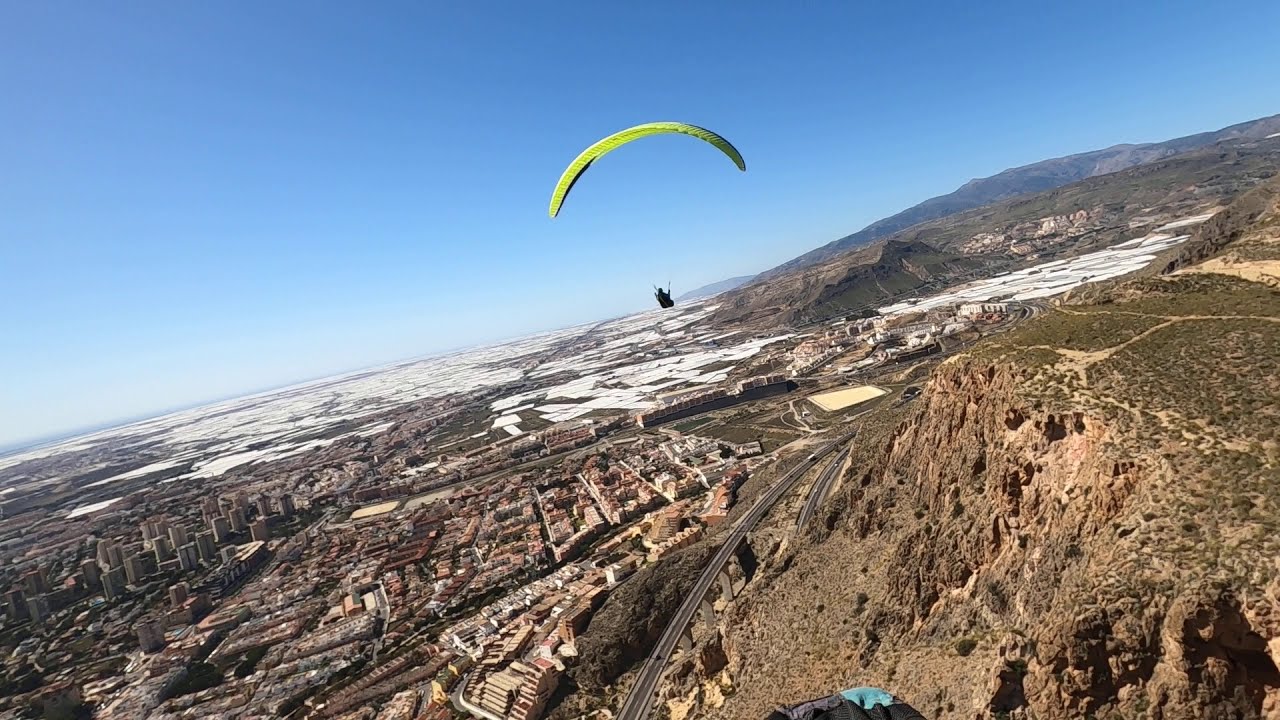The image showcases a high-altitude view of a hang glider hovering above a vast, arid valley with sparse greenery. The featured hang glider sports a bright yellow-green parachute and is positioned centrally, floating above a development that appears to be a city with a visible highway cutting through it. The landscape below is predominantly brown and rocky, with large cliffs and hints of snow in the distance, contrasting with grayish mountains in the backdrop. The sky above is a pristine, clear blue, enhancing the depth and breadth of the scene. Additionally, part of another hang glider is visible at the bottom of the image, suggesting the photo was taken from the perspective of another hang glider in the air.